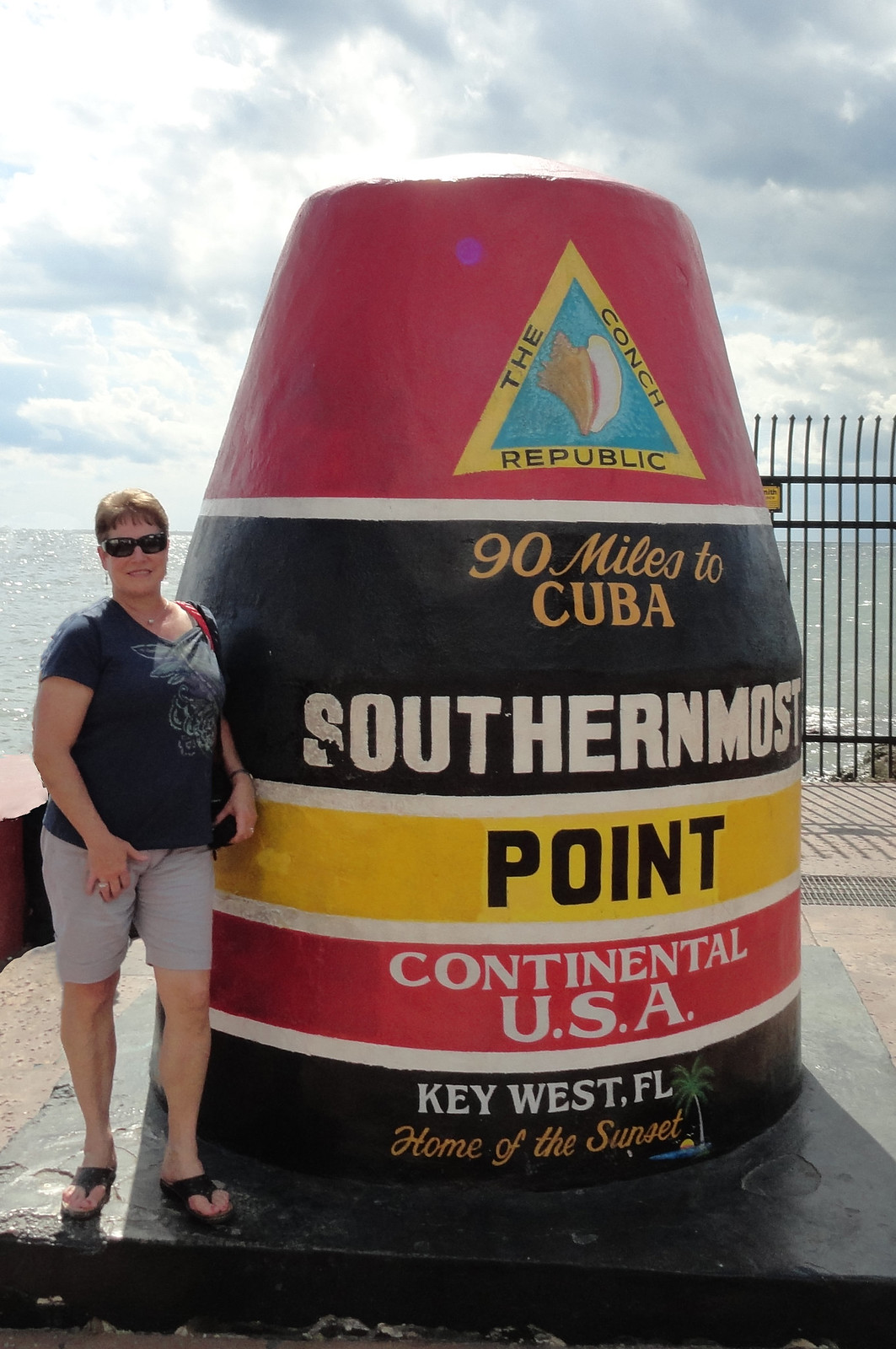This vibrant photograph captures a woman standing to the left of the iconic "Southernmost Point" buoy in Key West, Florida. The buoy itself is a striking concrete structure painted in bold colors: red, black, yellow, and white, with a small blue detail. It prominently features the text: "Conch Republic," "90 miles to Cuba," "Southernmost Point," "Continental USA," and "Key West, Florida, Home of the Sunset." The buoy is mounted on a black base and is adorned with a yellow triangle that encloses a blue interior and a drawing of a conch shell.

The woman next to the buoy is dressed in a dark blue short-sleeved shirt and gray shorts, with black flip-flops and sunglasses. She has peach skin and stands on a small platform directly to the left of the buoy, with the ocean behind her, showcasing the blue waters of the Gulf of Mexico. To the right of the buoy, a metal gate partially encloses the area. Above, the sky is a mix of blue and white with scattered clouds, setting a picturesque backdrop for this southernmost landmark known for its stunning sunsets.